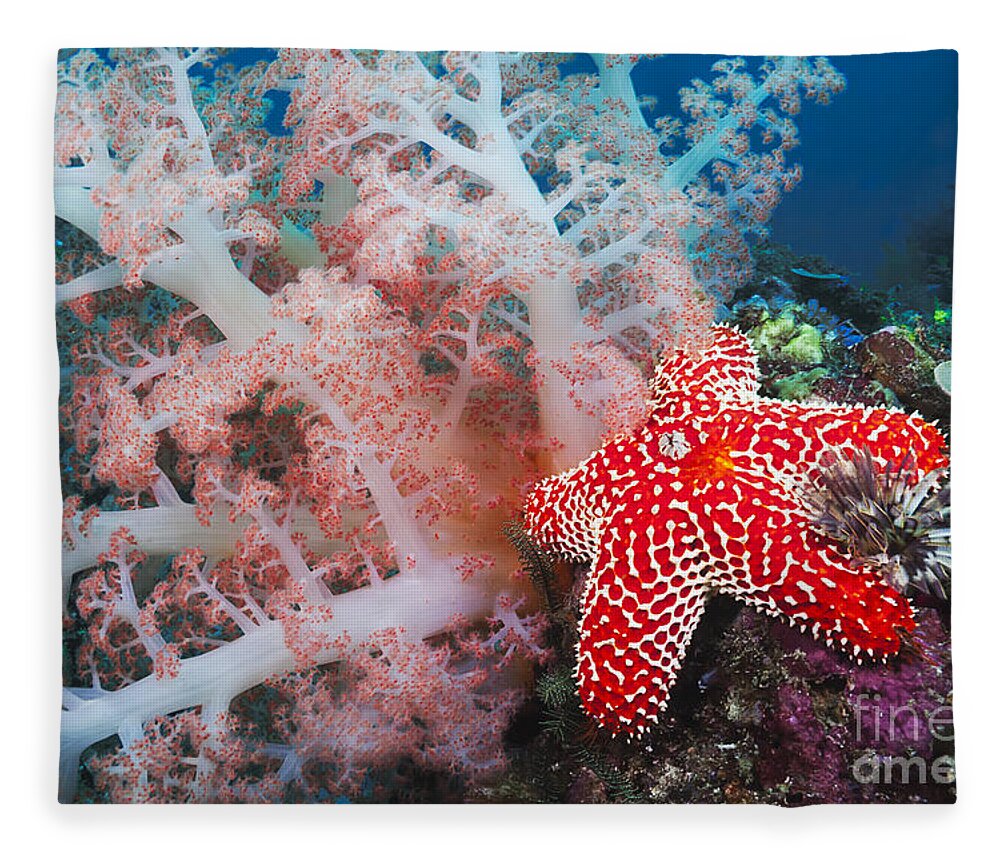This photograph captures a vibrant underwater scene in a natural ocean setting. At the center of the image is a large, healthy red starfish adorned with intricate white lines and web-like patterns, and featuring a hint of yellow at its center. The starfish is prominently placed on a rock-like formation that boasts shades of purple and green. To the left of the starfish, there's a striking sea plant or coral with white and pink hues, reminiscent of cauliflower but more loosely structured, with its buds speckled with red. The deep, tranquil blue of the water extends into the background, giving a sense of vastness. Additionally, in close proximity to the starfish, there is another distinctive sea organism that resembles a spiky sea urchin. In the bottom right corner of the photograph, there is partially visible text, which appears to include the words “F-I-N-E” and “A-M-E”.